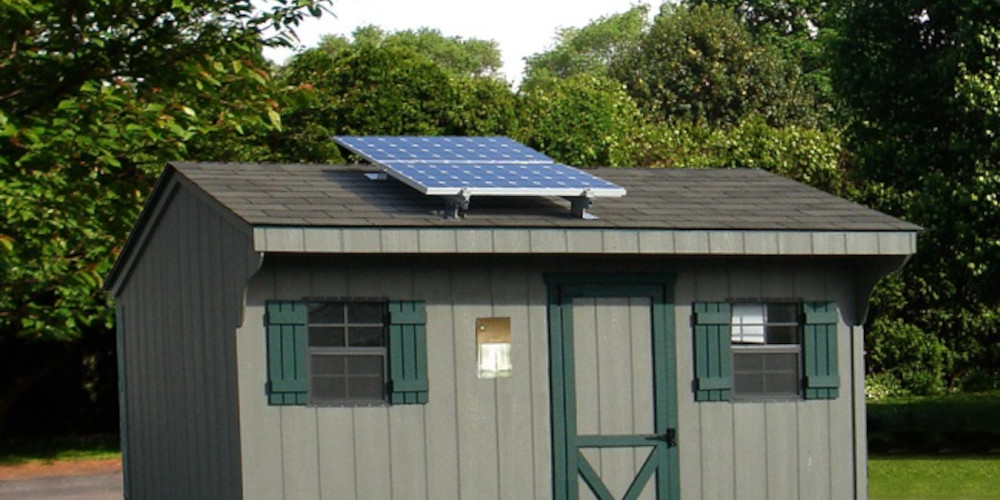This photograph captures a quaint backyard scene featuring a small, grayish-green shed with a dark gray shingle roof adorned with solar panels. The shed's exterior is constructed from wood paneling, characterized by horizontal planks in grey and olive hues. The dark green trim frames the barn-like door, which is secured with a black latch, adding a rustic touch to the structure. Flanking the door, on either side, are two small rectangular windows with dark green shutters detailed with vertical and horizontal slats. A sort of sign or note, possibly gold, is affixed to the wall between the left window and the door. At the lower part of the photograph, hints of grass, a driveway or asphalt, and some hedging are visible, though the image is tightly cropped, cutting off the view below two-thirds down the shed’s door. Behind the shed, a backdrop of tall green trees stands under a white sky, marking the serene, park-like ambiance of this setting.